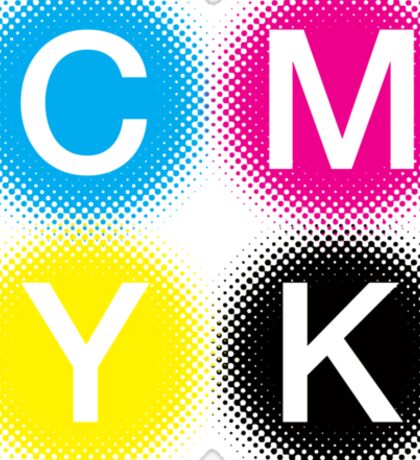The image features a white background divided into four quadrants, each containing a large white capital letter: C, M, Y, and K. In the top left quadrant is the letter C, backed by a dark sky blue circular color that fades into the white background using dots or a stippling effect. The top right quadrant has the letter M, which is set against a red-pinkish (fuchsia) circular background that similarly fades into white with dots. In the bottom left quadrant, the letter Y is positioned with a yellow circular background that transitions to white through stippling. The bottom right quadrant contains the letter K, fronted by a black circular color that also fades into white with dots. The stippling creates a blended effect where the colors gradually transition into the white background, giving a smooth gradient look. The precise, digitally rendered image ensures that all elements are evenly spaced and aligned within their respective quadrants.